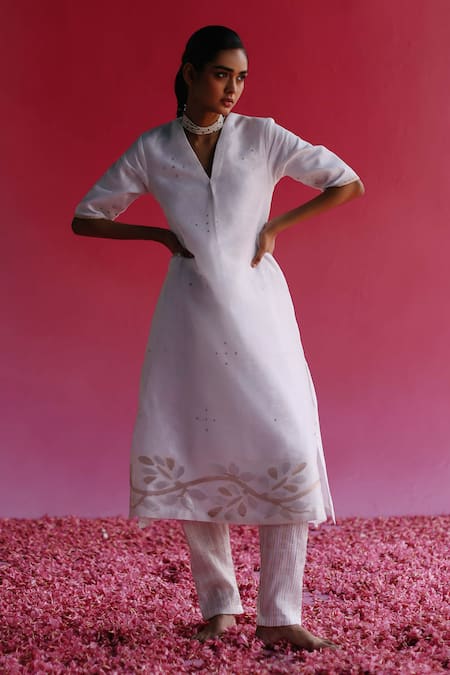The image captures a woman with a brown complexion, standing tall and proud with her hands on her hips, looking off to the right. She has dark hair styled in a ponytail and is dressed in a long, white dress that extends past her knees, featuring sleeves that reach her elbows. The dress is paired with faintly striped pants that go down to her ankles. A thick beaded white necklace adorns her neck. The bottom of the dress showcases a delicate pattern of branches with leaves. She is barefoot, standing on a bed of bright pink flower petals, which extends throughout the bottom of the image. The backdrop exhibits a gradient of pink hues, lighter at the base and deepening towards the top, complementing the vibrant petals on the ground.